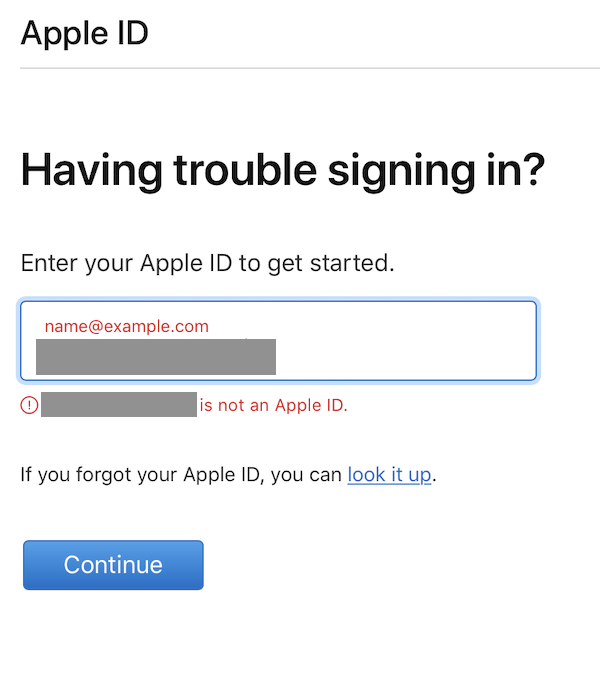This image features a simple design set against a white backdrop. In the upper left-hand corner, the word "Apple" is displayed, followed by the letters "ID". Below this, a gray bar extends across the width of the image. Beneath the gray bar, bold black text reads, "Having trouble signing in?"

Below this heading, additional black text states, "Enter your Apple ID to get started.". Positioned centrally is a white text box outlined with a double border - a dark blue inner line and a lighter blue outer line. Inside this box, placeholder text in red reads "Name@example.com", with the "@" symbol representing "at". The box's content appears to be blocked out by a gray overlay.

To the left of the text box, there is a red circle containing an exclamation point. Another gray block obscures additional text within this section. Adjacent to this, in red text, it declares, "Is not an Apple ID."

Further down, black text advises, "If you forgot your Apple ID, you can look it up." The words "look it up" are highlighted in blue, indicating a clickable link. Finally, a blue button at the bottom of the image contains the word "Continue" in white text.